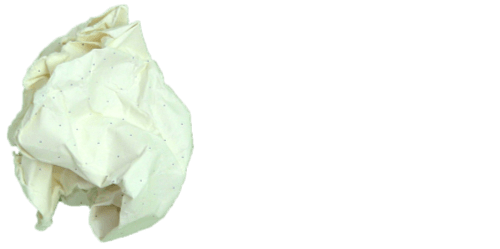The image depicts a blurry, crumpled piece of paper with a white, creamish to bluish tint, featuring small, uniform dots or specks scattered across its surface. The dots are either black or brown and arranged in an ordered, grid-like pattern, somewhat reminiscent of graph paper or a specially designed notebook page used for digitizing handwritten notes. The paper appears thick and somewhat elastic, possibly giving the impression of a child's diaper due to the crumpling. The background is largely nondescript, blending into the white of the paper, and shadows cast on the crumpled sections create subtle variations in color. The image as a whole appears more abstract and lacks clear definition, making it challenging to identify the exact nature of the object depicted.